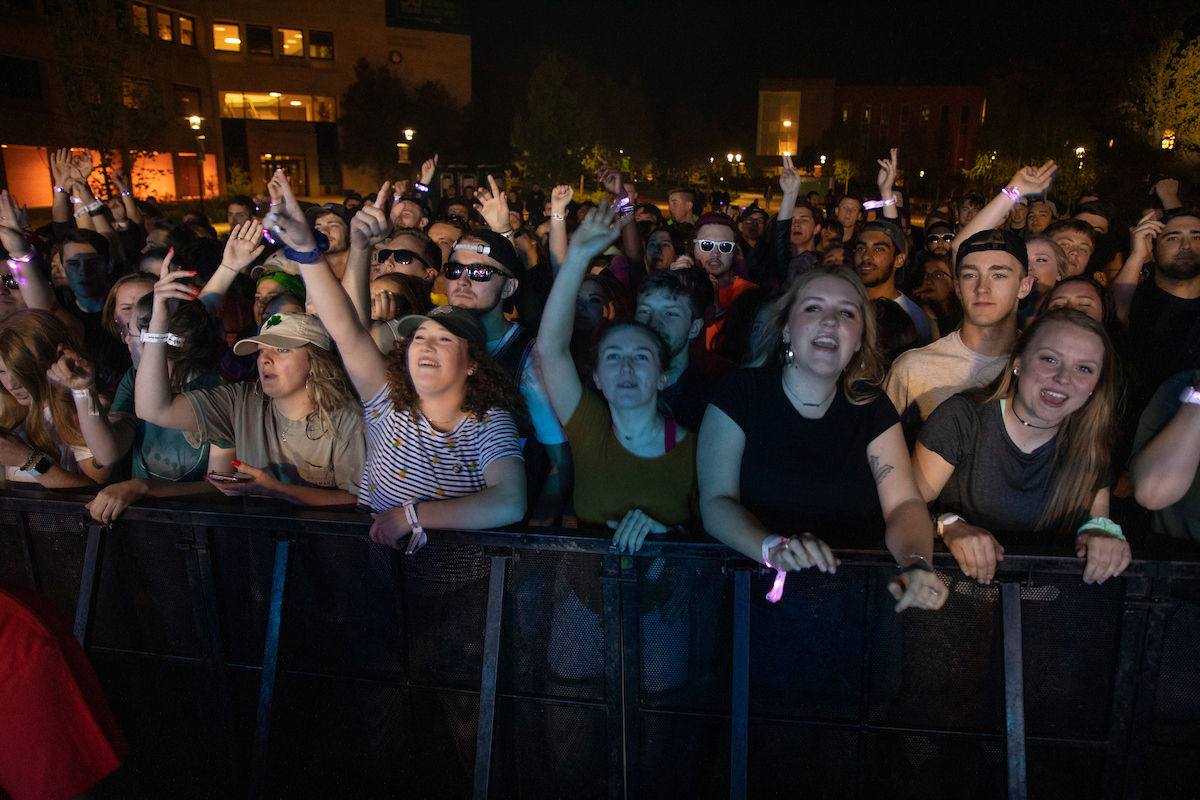This vibrant nighttime image captures a large, diverse crowd at an outdoor concert. The scene is brimming with energy as people relish the live music experience. In the foreground, an array of young concertgoers, predominantly women in the front row, stand tightly packed behind a black metal barricade. Many attendees have their hands raised, and a noticeable number are wearing sunglasses and wristbands, presumably from entry into the event. Smiling faces dominate the crowd, reflecting their enjoyment and excitement. The atmosphere appears warm, with attendees dressed in casual shirts. In the background, illuminated buildings, adorned with yellow lights shining through their windows, frame the bustling scene. Security personnel, identifiable by their red attire, also appear in the frame, ensuring the event runs smoothly.